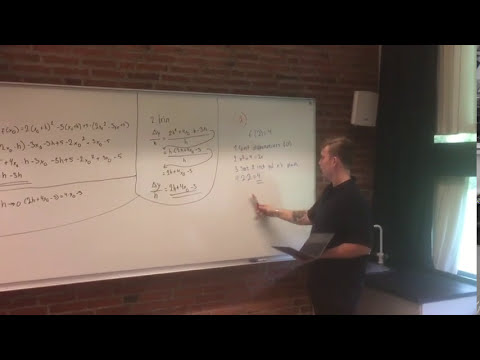The image captures a detailed scene of a teacher in a classroom. The classroom has red brick walls with a whiteboard mounted on one of them. The teacher, wearing dark clothing consisting of a black polo shirt and black pants, stands in front of the whiteboard. He has short brown hair and visible tattoos on his right arm, which is holding a marker. His left hand holds an open book or possibly a laptop. To his side, there's a sink and on the far right, there are windows with curtains.

The whiteboard is filled with various equations and numbers, divided into three sections by lines. The teacher appears to be focusing on the rightmost section of the board. His side profile suggests he is actively engaged in explaining the content. A marker lies on the tray attached to the whiteboard, indicating it's an ongoing lesson. Though the exact subject is unclear, it likely involves math or a scientific topic. The classroom ambiance hints at an interactive and attentive learning environment, even if the students are not visible in the image.